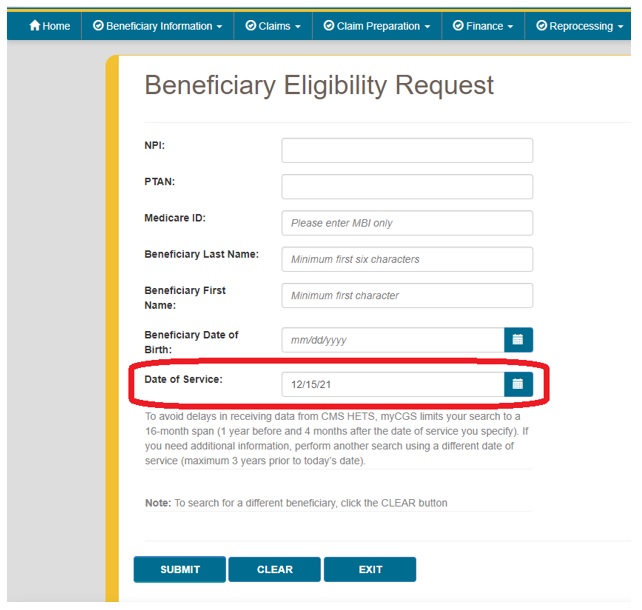The image displays a detailed interface of what appears to be an insurance website. At the top, there is a prominent green banner. The website is organized into several categories, each represented by icons and text. Starting from the left, there is a home icon accompanied by the word "Home." Next to it is a circular icon featuring a checkmark, labeled "Beneficiary Information," which is a drop-down menu. Following that, there are additional circles with checkmarks for further drop-down menus labeled "Claim," "Claim Preparation," "Finance," and "Reprocessing."

In the center of the page, a notable rectangular section bordered by vertical yellow lines and a thin horizontal yellow line stands out. This section carries a bold heading in large black letters that reads "Beneficiary Eligibility Request." Below the heading, the section is subdivided into several labeled rectangles aligned on the left-hand side. They are labeled as follows: "MPI," "PTAN," "Medicare ID," "Beneficiary Last Name," "Beneficiary First Name," "Beneficiary Date of Birth," and "Date of Service." The "Date of Service" field is conspicuously outlined in red to highlight its importance.

At the bottom of the section, there are three buttons labeled "Submit," "Clear," and "Exit," providing options for user interaction. The detailed structure and highlighted elements suggest that this is a functional interface for processing beneficiary information on an insurance platform.